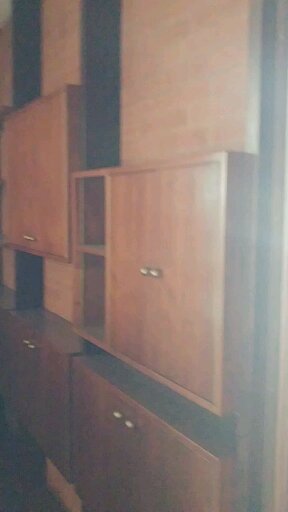The image features what appears to be a section of a living room embellished with a brick wall. Centrally placed against this wall is a detailed wooden cabinet, constructed from natural wood, lending it an authentic and expensive appearance. The cabinet is composed of several distinct sections. 

On the lower level, there are two side-by-side storage units featuring doors with gold or bronze handles that open forward. Above the left of these units, a similar storage piece is positioned lifting upwards, with light brown or bronze handles at the bottom. To the right, situated higher up, there's another box-like compartment with two doors that open outward, revealing internal space divided by shelves.

On the left side of the cabinet, there appear to be vertical strips, possibly black, adding contrast to the predominantly wooden structure. The perspective of the image suggests that the right side is closer to the viewer, with the cabinet structure receding to the left, emphasizing the room's depth. The intricate detailing of the woodwork with strategic brass or gold-toned handles and the cabinetry’s integration into a brick wall – which appears to have sections and spaces, creating an intriguing visual effect – all contribute to the room's sophisticated and warm ambiance.